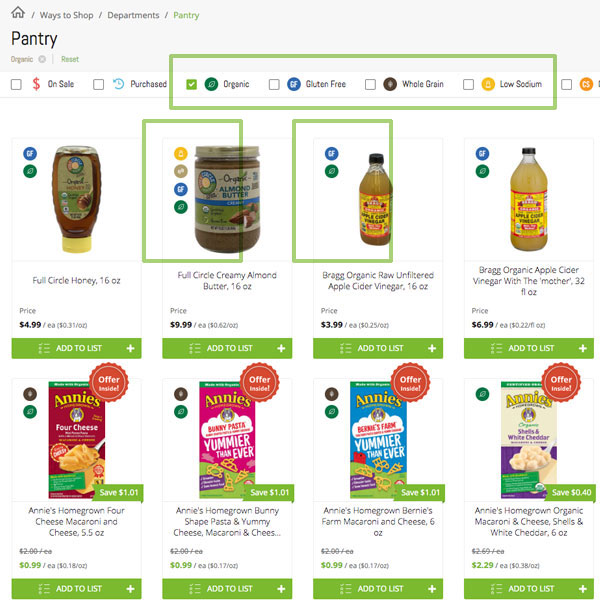This image features an organized layout on a white background, with different sections and product listings, suitable for an online grocery shopping interface.

At the top section, there is a thick blue bar, containing a small black house icon, followed by navigational elements separated by lines: "Ways to Shop," "Departments," and "Pantry."

Below the bar, the focus shifts to a "Pantry" section, marked by categories such as "Organic" with a reset option symbolized by a small circle with an 'X'. A subsequent white box holds functional icons: a tiny blue box with a red dollar sign indicating sales, another blue box with a clock and arrow for purchased items, followed by a larger green block emphasizing organic products. Within this green block are smaller green boxes with check marks, labeling foods as "Organic," "Gluten-Free," "Whole Grain," and "Low Sodium."

Outside this green block is an orange circle with further categorization, followed by the start of the product listings.

1. **Full Circle Honey (16 ounces) - $4.99**: This listing includes a blue circle with a shopping cart icon and a green circle with an unspecified icon, along with a green "Add to List" button at the bottom.

2. **Full Circle Creamy Almond Butter (16 ounces) - $9.99**: Highlighted by a green square, this product also features a yellow, purple, blue, and green circle, with the "Add to List" option provided.

3. **Bragg Organic Raw Unfiltered Apple Cider Vinegar (16 ounces) - $3.99**: This listing includes green and blue circles along with the "Add to List" button.

4. **Bragg Organic Apple Cider Vinegar with the Mother (32 fluid ounces) - $6.99**: This item also contains green and blue circles and an "Add to List" button.

5. **Annie's Homegrown Four Cheese Macaroni and Cheese (5.5 ounces) - $0.99**: Marked down by $1.01, this product has a green flag indicating savings and a red circle noting "Offer Limited", complemented by brown and green circles and an "Add to List" button.

6. **Annie's Homegrown Bunny Shape Pasta and Yummy Cheese Macaroni and Cheese (5.5 ounces) - $0.99**: Similar to the previous item, it offers $1.01 in savings, carries an "Offer Limited" red circle, brown and green icons, and an "Add to List" option.

7. **Annie's Homegrown Bernie's Farm Macaroni and Cheese (6 ounces) - $0.99**: Another marked down product with a $1.01 savings, an "Offer Limited" red circle, brown and green icons, and an "Add to List" button.

8. **Annie's Homegrown Organic Macaroni and Cheese, Shells and White Cheddar (6 ounces) - $2.29**: Boasting a 40 cent saving and an "Offer Limited", accompanied by a green box and an "Add to List" button.

The meticulous details and color-coded elements help users navigate and select their desired grocery items efficiently.